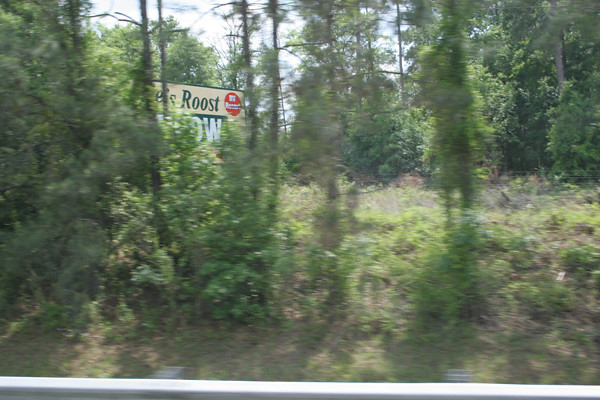This photograph captures a roadside view, seemingly taken from within a car, as evidenced by the faint edge of a car window visible at the bottom of the frame. The scenery beyond the car window reveals a dense woodland area, characterized by a mixture of hardwood and pine trees. Vines are seen climbing some of the tree trunks, while light filters through the leafy canopy, creating a serene, dappled effect. On the left side of the photo, partially obscured by the trees, stands a rectangular billboard. The background of the billboard is beige, and though the entire text isn't visible, it prominently features the words "Something's Roost" and "9W" in large green letters. Adjacent to the word "roost," a red label with white text appears to read "RV Resort." This subtle amalgamation of natural and human elements conveys a quiet, roadside environment gently interrupted by signs of civilization.